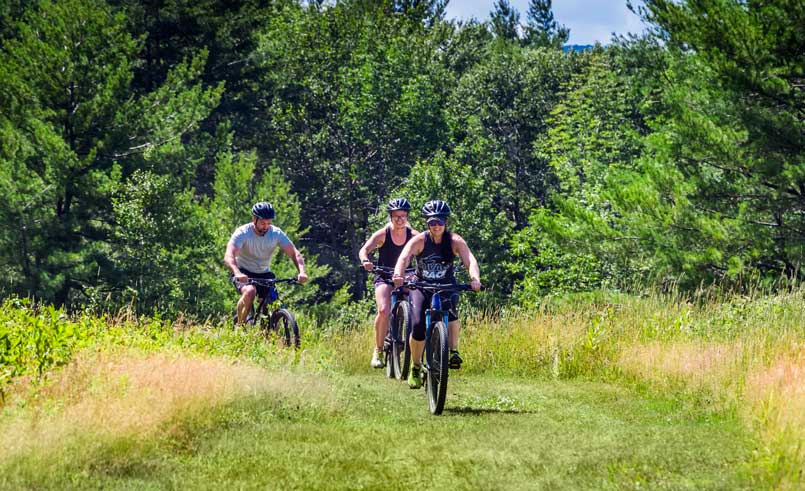This vibrant outdoor photograph captures three mountain bikers on a grassy trail in a wooded area under a bright blue sky. The riders, two females in black tank tops and shorts and a male in a gray t-shirt and shorts, all sport blue helmets as they pedal towards the photographer. The trail, composed of short green grass interspersed with brown tufts and other vegetation, is flanked by taller grass and wild flora. In the background, dense green trees stretch toward the horizon. The lively movement of the bikers, with their dark bicycles accented with blue trim, adds dynamic energy to the scenic, sunlit setting.